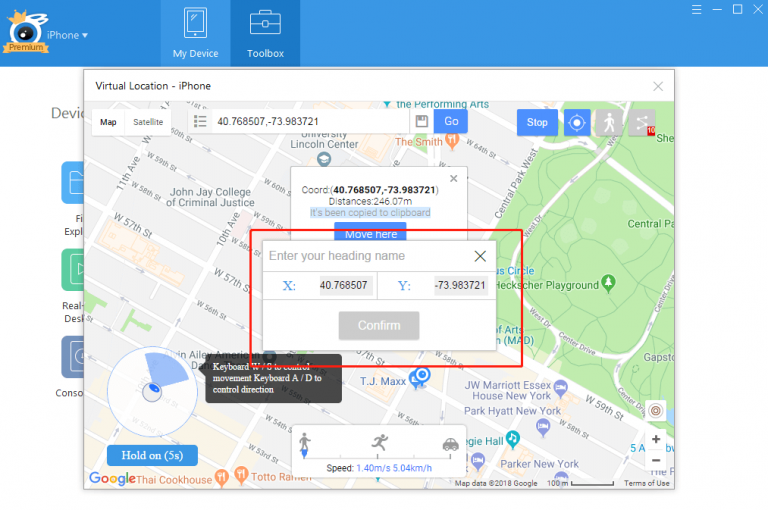The top of the image features a blue border with a central icon consisting of three concentric circles: black, blue, and white. Above the circles is a gold crown, and below them, a gold banner with the word "Premium." 

Beneath this header, there is a drop-down menu labeled "iPhone" followed by three buttons: "My Device," "Toolbox," and a blue screenshot from Google Maps titled "Virtual Location iPhone." The map view displays two options: "Map" and "Satellite." An associated box shows the coordinates 40.769507, -73.983721, alongside a blue "Go" button.

Further down, there is a white box surrounded by a red rectangular border. Inside the white box, it prompts users to "Enter your heading name" and displays two fields: one marked with a blue "X" containing the value 40.768507, and another marked with a blue "Y" showing -73.983721. At the bottom of this section, there is a gray "Confirm" button.